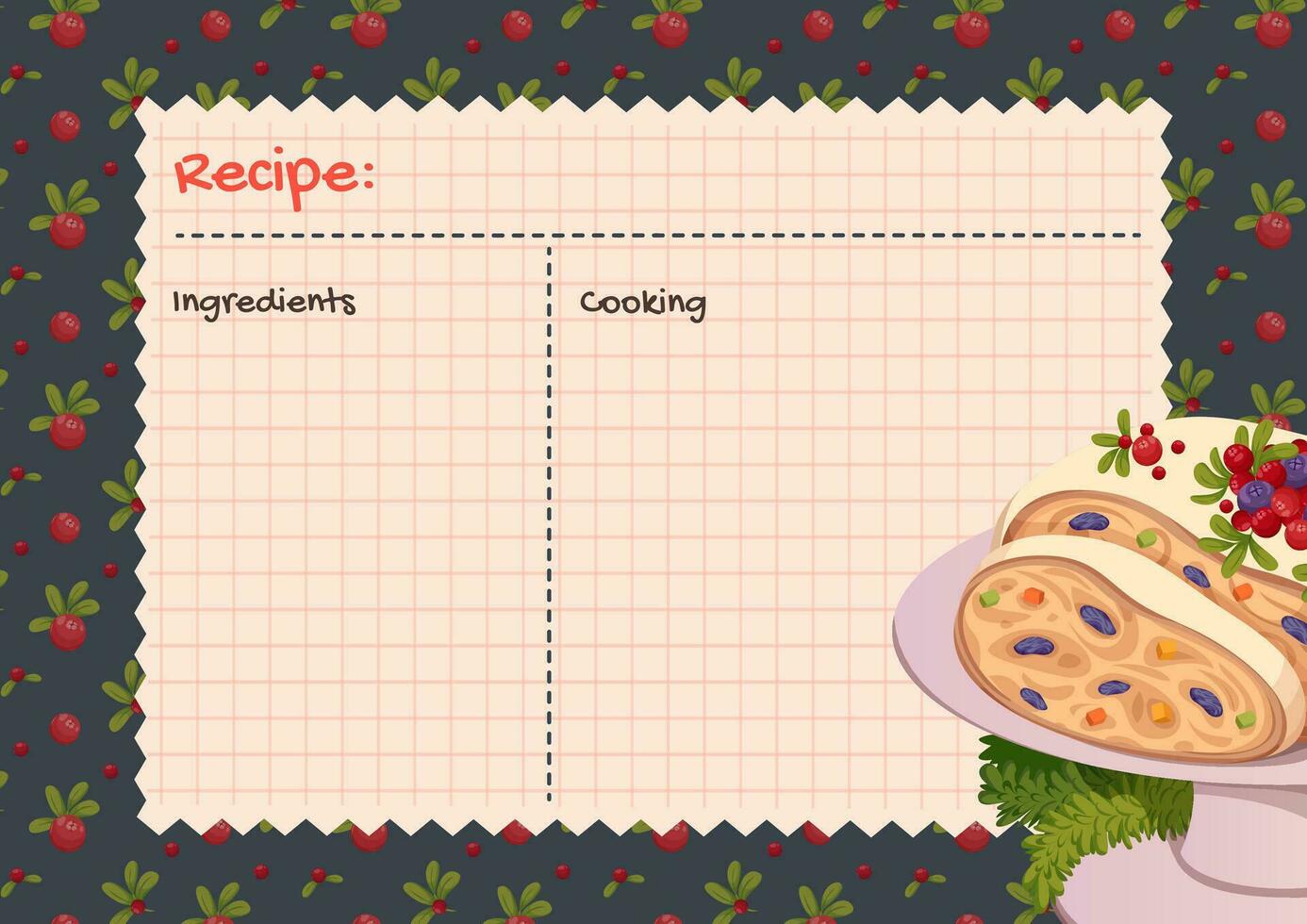This image is a horizontally aligned, rectangular design meant for creating a recipe. The background features a dark gray color adorned with numerous small strawberries and green leaves, creating a border-like effect around the edges. Centrally, there is a tan, grid-patterned rectangular shape with slightly darker grid lines. The upper left corner of this central shape prominently displays the word "Recipe" in orange followed by a colon, beneath which runs a dotted line extending across the width. Another dotted line vertically divides the grid into two sections: the left column labeled "Ingredients" and the right column labeled "Cooking," both titles in black text. Additionally, in the lower right corner of the image, there's an illustration that appears to depict a platter of bread with dried fruit, though it could also resemble a bonnet or hat due to the presence of what seems like a neck and shoulder beneath it. The overall design is intended to be downloaded and personalized with specific recipe details.